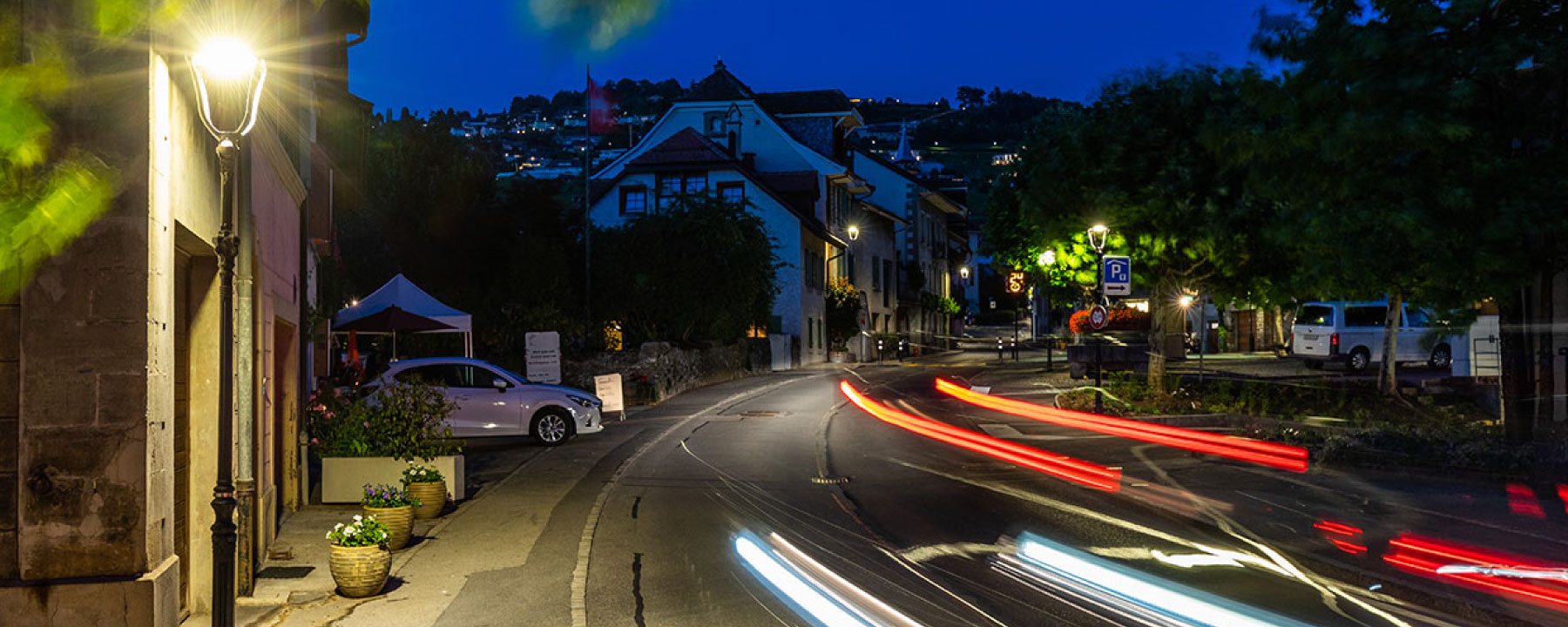The photo captures a well-lit, futuristic-looking town at night, featuring a winding street that curves from the lower right to the center and then back to the right. On the left side of the street, there is a mix of concrete buildings, including one with a doorway, adorned with three concrete flower pots filled with white and purple flowers. Above it, a tall, illuminated street lamp stands out. Further down, there's a small white tent and a car poised to pull out into the street. The right side of the street is lined with large trees brimming with green leaves, a rock wall with shrubbery, and various houses including a two or three-story white house. Noteworthy elements include a blue parking sign with a "P" and arrow, a no parking sign, and a white van parked in a driveway. The foreground features striking red and white light streaks, presumably from a time-lapse capture of vehicle taillights and headlights, adding to the street's modern and dynamic atmosphere. In the background, a hill dotted with houses rises against the dark night sky, illuminated by streetlights on both sides of the street below.